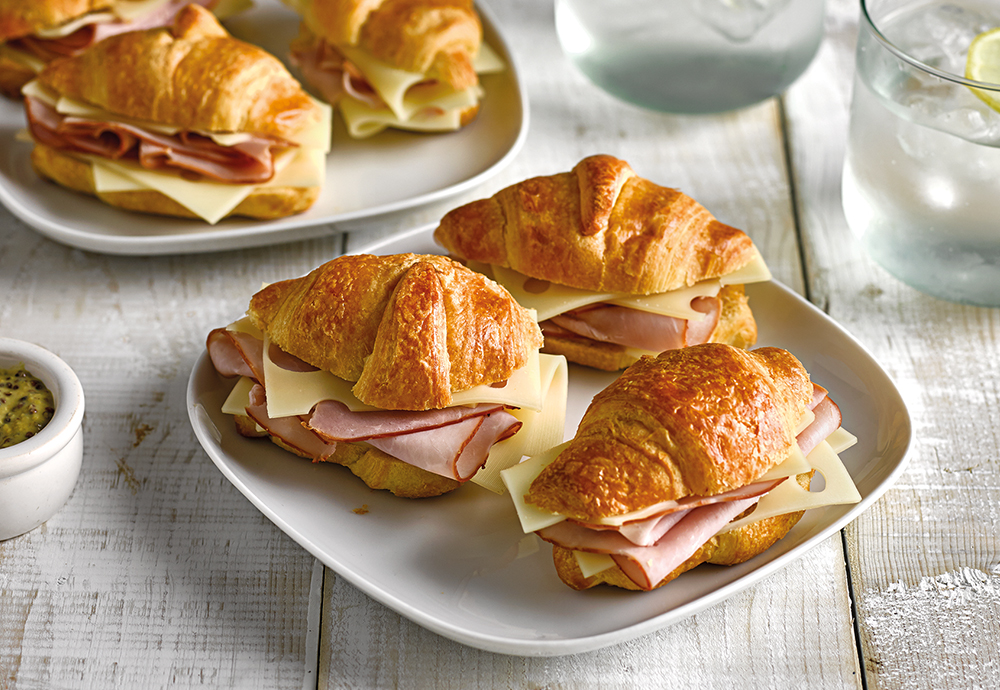In this detailed photograph, the main focus is a white, round-edged square plate centered slightly towards the bottom, holding three croissant sandwiches filled with Swiss cheese and ham. Each sandwich is meticulously placed: one at the bottom right, another slightly above to the left, and the last one in the upper right corner. The plate sits on a light gray, rustic wooden table that looks as though it's been painted white. Adding to the rustic composition, another similar plate of croissant sandwiches extends out of the frame at the top left corner. To the left of the main plate, a small white ceramic bowl containing a green and yellow mixture is partially visible off the edge of the image. Above and a touch to the right of the main plate, there’s another white bowl that also extends off the image. Nearby, a clear glass of water with a lemon slice is positioned just out of the frame on the top and right sides. The entire scene exudes a casual, yet carefully arranged, culinary display on a weathered wooden surface.